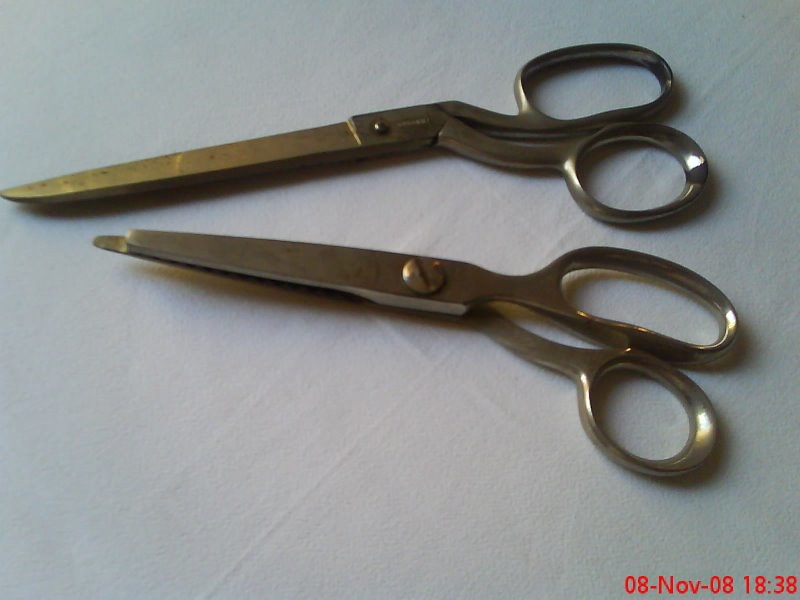This is a detailed photograph of two pairs of heavy-duty, metal scissors, prominently displaying their aged and rusty appearance. They lie on a white background, which might be paper or fabric but appears soft in texture. The image captures a historical feel, emphasized by the date stamp in the bottom right corner, marked "08-NOV-08" with a time notation "1838." The scissors differ in both design and condition: the pair in the foreground features a broken tip, while the pair in the background has an angled blade. They are right-handed scissors, each displaying distinct characteristics despite their overall similarity. A subtle light illuminates the right side of the scissors, accentuating their metallic surfaces and separating the handles slightly while both cutting edges point leftward.